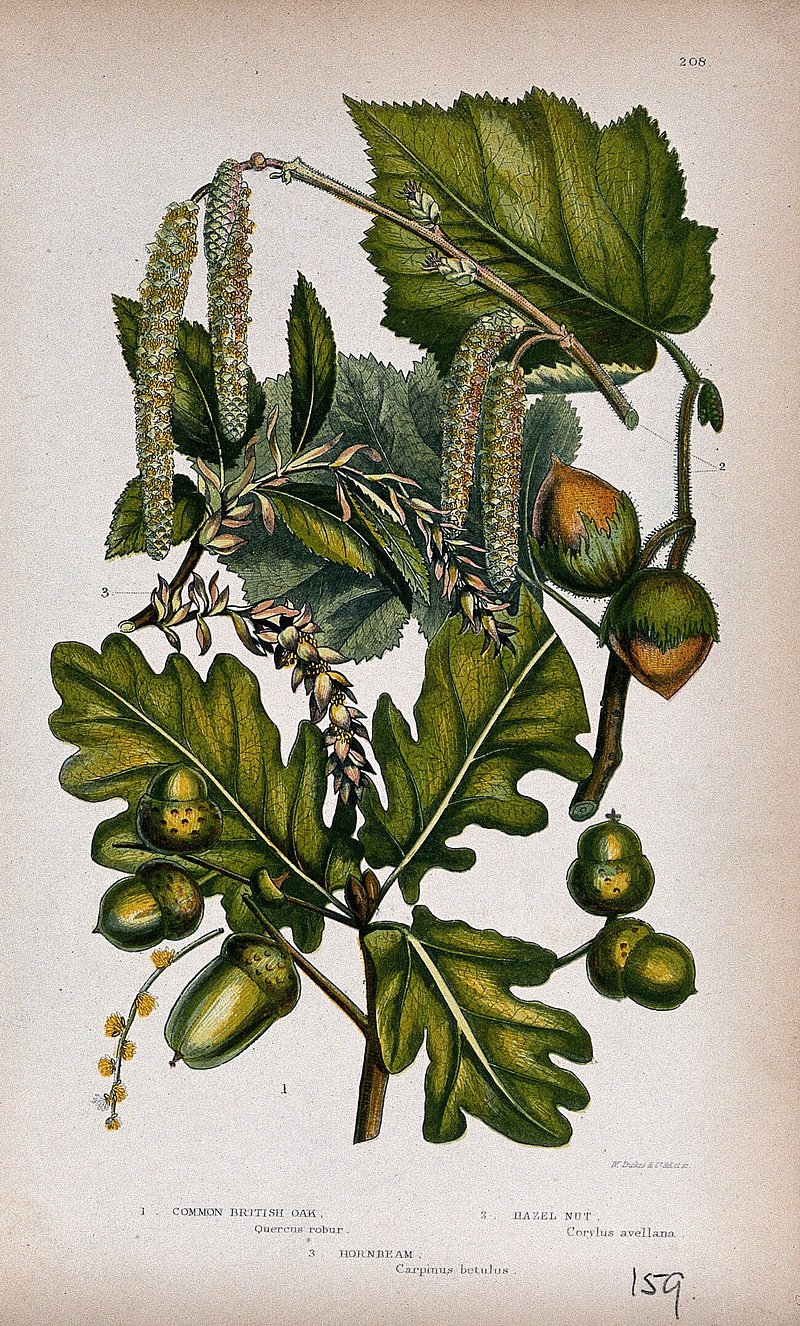The image depicts a detailed, vintage botanical drawing of a plant, likely modeled after a real specimen. The main plant structure comprises green leaves of various shapes and sizes, with branches extending in multiple directions. The drawing features intricate details including prickly hair-like projections along the vines. Different elements such as acorns, yellow bulbs with green caps, and other nut-like forms are depicted on the branches, showcasing parts of the plant that might be found in nature. This botanical illustration appears low in saturation with colors including green, orange, yellow, and tan. Labels in a small, typewriter-like font identify the plant parts, despite being difficult to read. The text specifies the names "common British oak," "hazelnut," and possibly "hornbeam," with an indication of scientific nomenclature. There is also a handwritten number "159" on the lower right side of the parchment-like, cream-colored background.